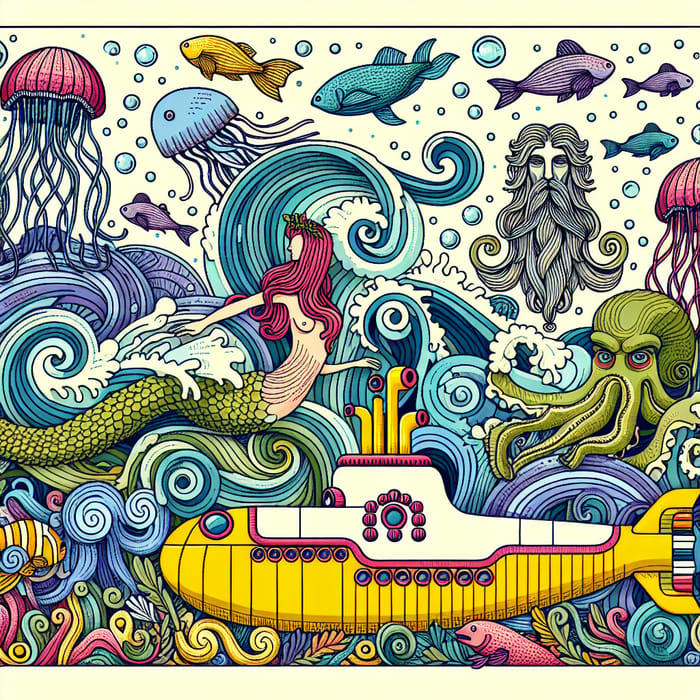The image depicts an underwater scene filled with vibrant colors and a variety of aquatic life, resembling a whimsical painting or cartoon collage. Central to the scene is a yellow submarine with a white top and pink windows, reminiscent of the iconic Yellow Submarine by Drumroll Beetle. Surrounding the submarine are diverse sea creatures, including jellyfish, squids, an octopus, and numerous fish in shades of yellow, blue, purple, and violet. Dominating the scene is a mermaid with long, pink hair adorned with flowers, and a green fish-scale tail. She is topless with her upper body visible, adding an element of classic mermaid mythology. Intricate water waves, composed of individual lines in blue, white, and purple, weave through the scene. Among the figures is also an old man with a long beard and hair, reminiscent of Poseidon, adding a mythical element. Colorful water plants in yellow, pink, and green add to the lush, fantastical environment, making this artwork a visually striking piece that seamlessly blends various underwater elements into a cohesive, imaginative tapestry.